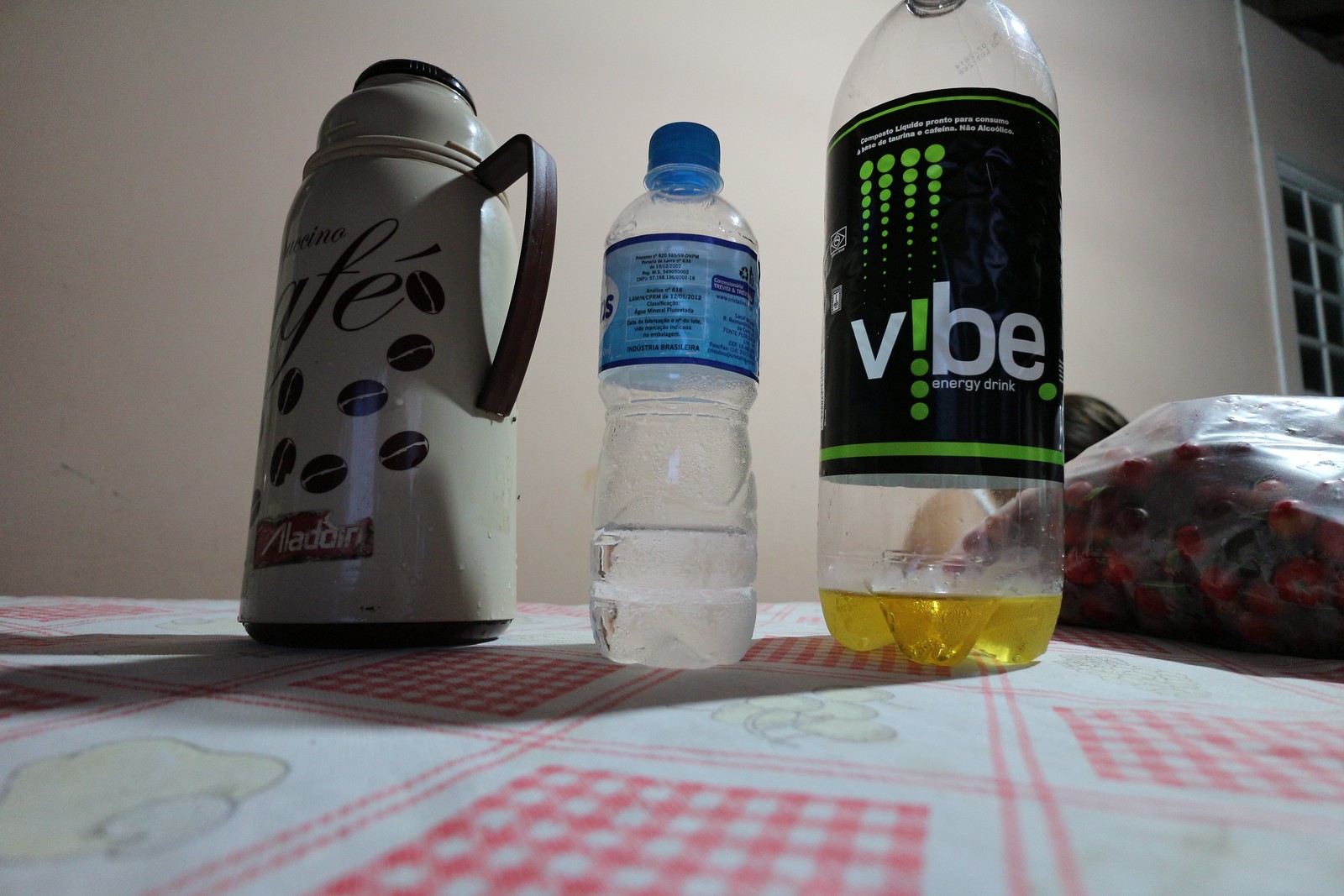This is a detailed color photograph of a table featuring three distinct drink containers set against a red and white checkered tablecloth with a subtle patterned art print. The tablecloth exhibits a traditional checkerboard style, segmented by double red lines. In the background, there is a light-colored wall with a visible window on the right side, adding a domestic feel to the image.

On the far left, a gray thermos with a black handle and lid prominently displays the word "CAFE" in black lettering alongside various depictions of coffee beans. Beneath it, a partially worn label reads "ALADDIN," signifying the brand.

The centerpiece of the arrangement is a clear plastic water bottle, approximately a quarter full, marked with a blue cap and a partially visible blue label. The back of the label is facing the camera, so the brand remains unidentified.

To the right of the water bottle stands a nearly empty Vibe energy drink bottle. This tall container features a black label with fluorescent green accents and the word “VIBE” prominently displayed in white text. A small amount of yellow liquid remains at the bottom of the bottle.

Additionally, behind the Vibe bottle, a clear plastic bag filled with what appears to be cherries or a similar red fruit can be seen partially, adding a touch of color and texture to the scene.

The composition is captured from a low-angle perspective, almost level with the table surface, providing an even view of the bottoms of the bottles and accentuating the detailed textures and colors of both the objects and the tablecloth.